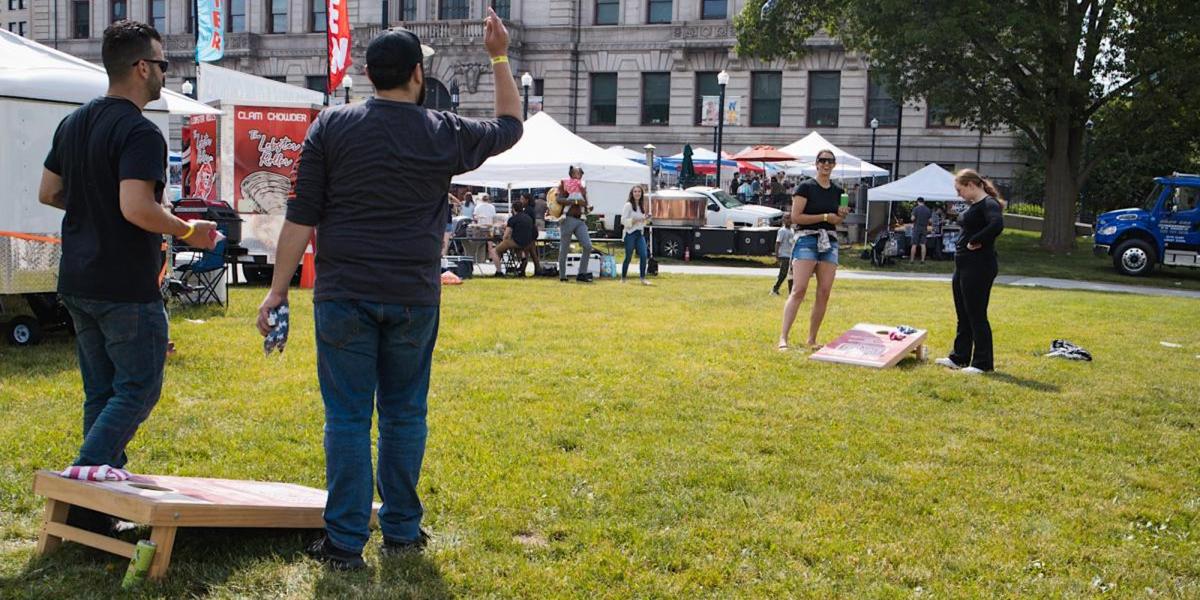The photograph captures a vibrant outdoor event styled as a park gathering. In the foreground, four people, split into two groups, are engaged in a lively game of cornhole on a green lawn. On the left, two men, both in jeans and dark shirts, participate in the game, with one man sporting a hat and preparing to toss a bean bag. To the right, two women, one in jean shorts and a short-sleeve shirt and the other dressed in all black, are enjoying the game, with the woman in sunglasses laughing heartily. The setting suggests a festival or a farmer's market, indicated by multiple white canopy tents and vendors scattered around the courtyard in the background. Notably, a large beige stone building with rectangular windows and a tree stands majestically to the right side of the image. Additional onlookers and a blue truck can also be seen further enriching the scene. The overall atmosphere is one of community and fun under the open sky.